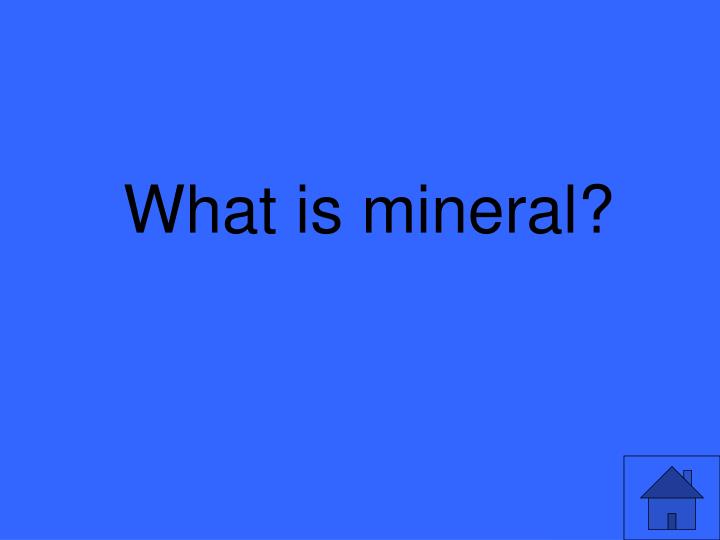The image features a vibrant blue background, slightly darker than sky blue but bright and rich in color. Prominently positioned just above the center in large black letters, the text reads "What is mineral?" with a capital 'W' and a question mark. In the lower right corner, there's a simplistic clipart illustration within a thin black-outlined square. This illustration depicts a basic house, comprising a rectangular body, a dark gray triangular roof, a single door, and a small chimney on the right side of the roof. The overall design exudes simplicity, resembling a slide from a PowerPoint presentation.